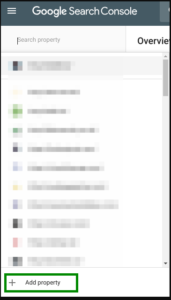This image depicts a screenshot that is heavily blurred, rendering most of its content illegible. However, the background is identifiable as Google Search Console, characterized by its classic white interface. Centrally highlighted, a green rectangle frames the option labeled "Add Property," drawing attention amidst the overall blurriness. The surrounding elements remain indistinct, making the outlined "Add Property" function the primary focal point of the image.